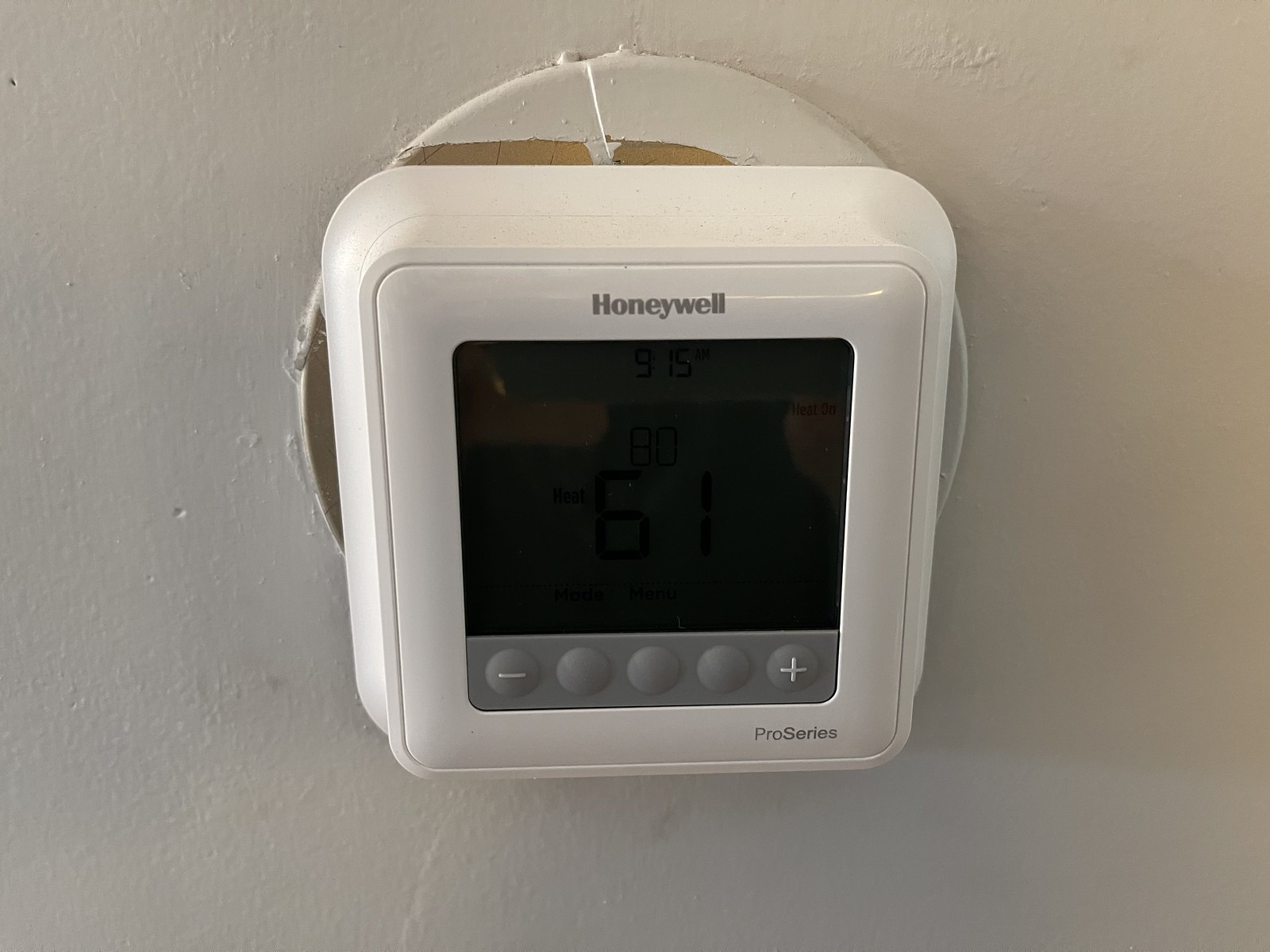The image depicts a rectangular, photographic picture featuring a white wall as the background. Centrally mounted on the wall is a white temperature monitor, identified by the brand name "Honeywell" in gray letters at the top. The temperature monitor is attached to a circular fixture with brownish hues visible behind it. The monitor displays a black screen with important information: the time reading "9:15," the current temperature of "80," and the heating setting at "61," all shown in black. The device includes gray buttons on both sides—a minus button on the left and a plus button on the right. Additional text "Pro Series" is also visible in gray on the monitor.